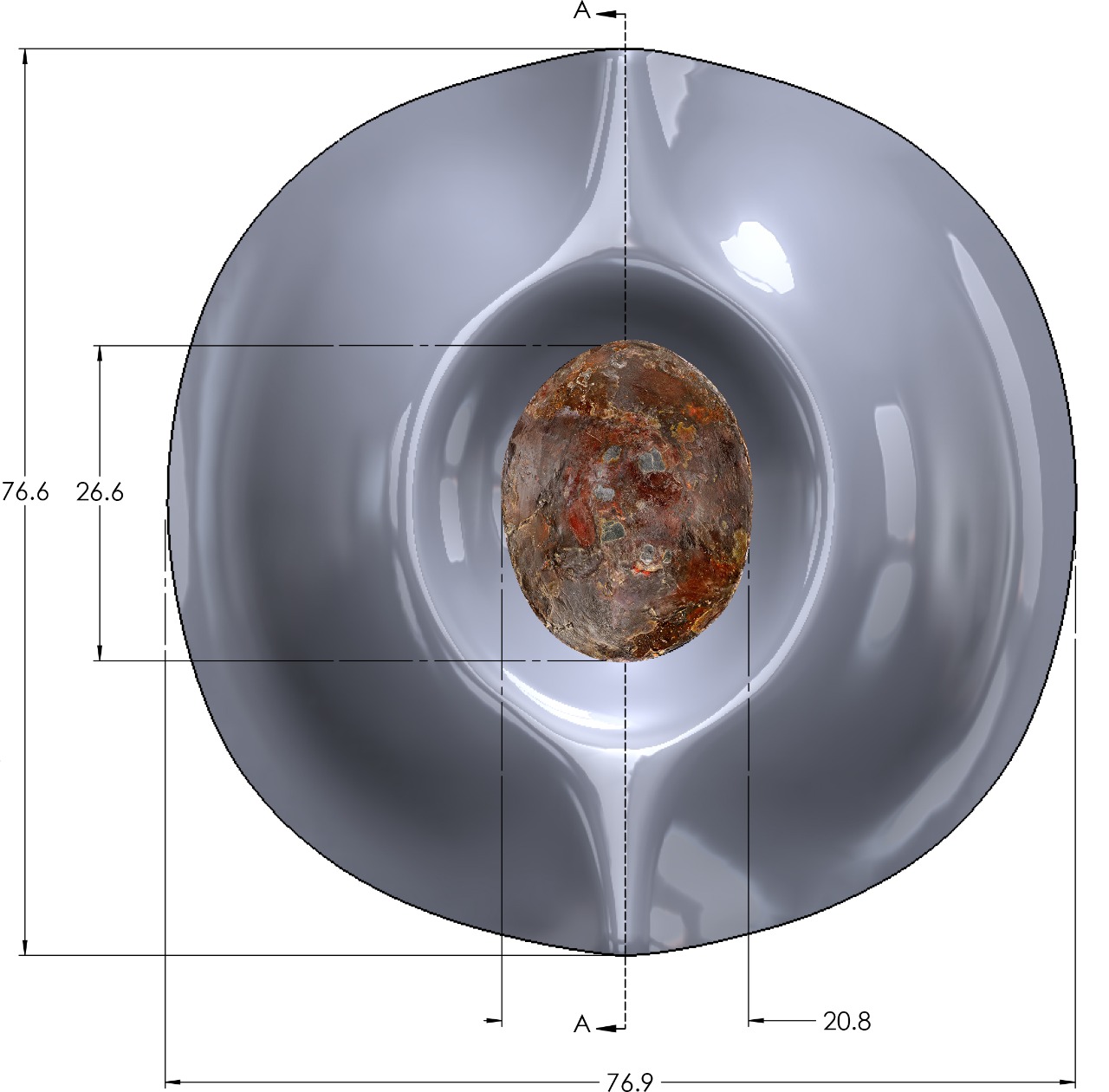The image depicts a round, grayish object with a shiny surface, resembling either a plastic or metallic material. The object has a prominent depression at its center, reminiscent of a geological cut revealing crystal formations. The central depression contains multicolored, possibly abstract elements that evoke the appearance of dark flowers or crystalline structures. Surrounding the object is a series of tiny squares with numerical measurements, including labels such as 'A', 'B', 76.6, 26.6, 76.9, and 20.8, suggesting it could be a design or prototype with precise dimensions. The background is pure white, emphasizing the object without any additional distractions. The detailed annotation indicates the image might be instructional, possibly conveying the object's specifications for replication or study.